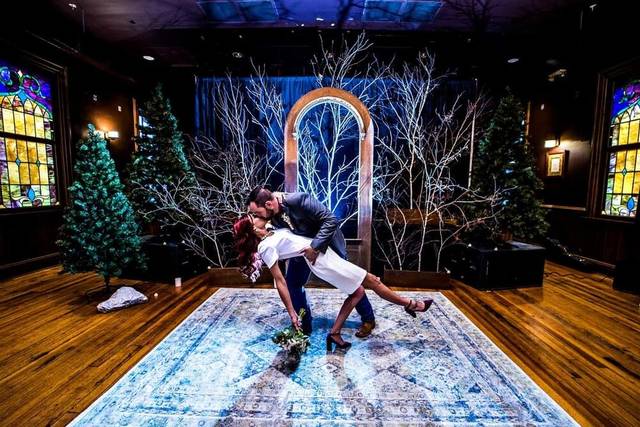The image captures a tender moment where a wedding couple is dancing in a richly detailed indoor setting. The groom, a Caucasian man with dark hair and a full beard, wears a dark blue suit with brown shoes, holding his bride in a graceful dance dip. The bride, also Caucasian, has dark hair and dons a short white dress and black high-heeled shoes, while clutching a bouquet of flowers in her right hand. She leans back with her left leg extended, supported by the groom’s strong embrace around her waist and shoulders.

Their intimate moment takes place on a vibrant blue patterned dance floor, surrounded by a warm hardwood floor. Behind them, the room is adorned with an eclectic mix of decor, including a painting of a winterscape with naked-branched trees, and various pine-like evergreen decorations signifying a Christmas theme. Large stained-glass windows frame the scene on the left and right sides, contributing to the church-like atmosphere. The ceiling features wooden beams with soft, recessed lighting, completing the cozy ambiance. The backdrop of the photograph reveals an archway, further layered with the winter-themed decorations, highlighting the festive and romantic setting of this cherished moment.